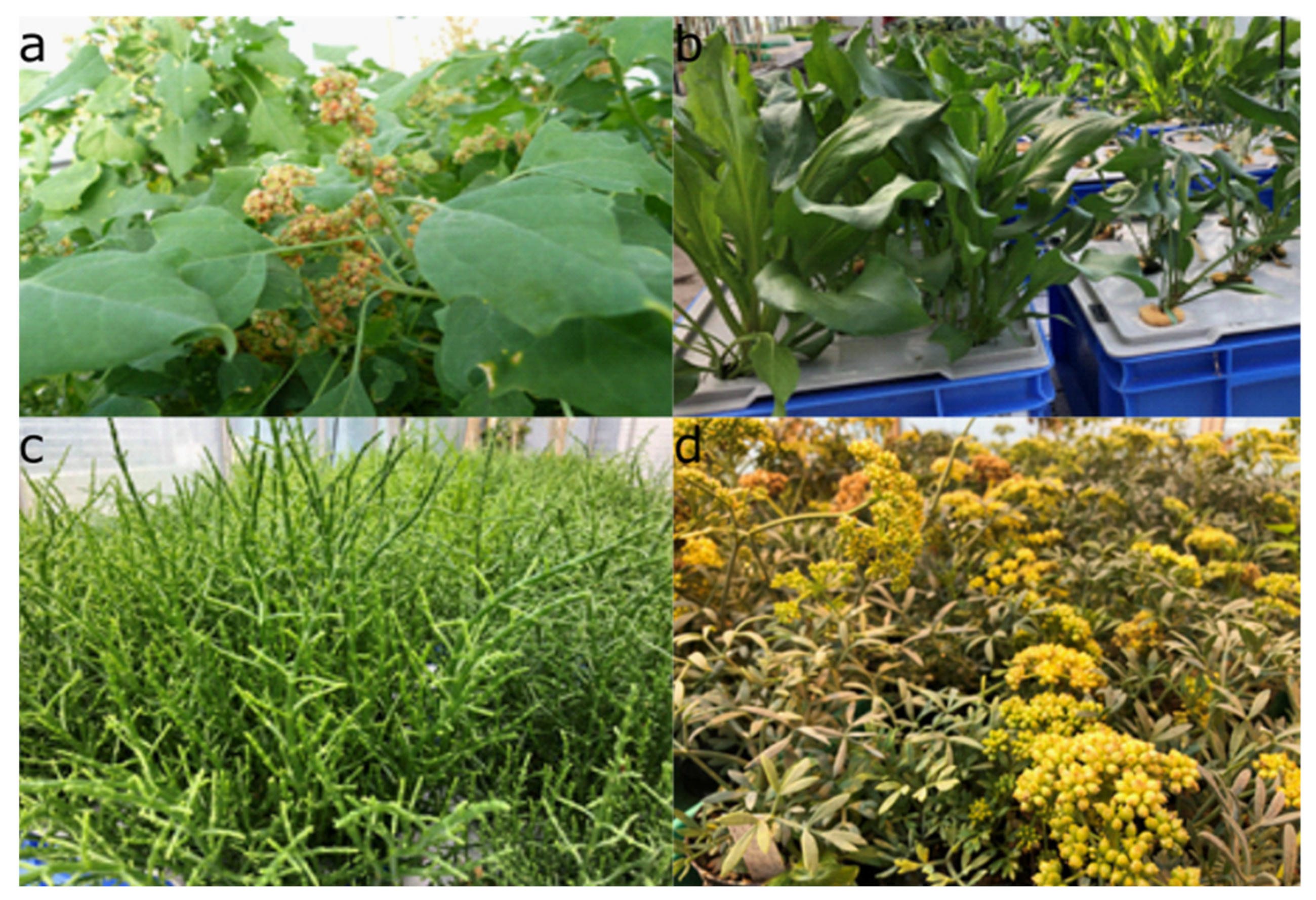The image is a quad-photo collage labeled A, B, C, and D, featuring detailed close-ups of various plant types in different settings. At the top left, picture A showcases a large leafy green plant with small white-tannish seed pods or flowers concentrated in the middle. Moving to the top right, picture B features tropical indoor plants thriving in blue and white planters arranged in a greenhouse environment. These plants appear to be emerging through perforated lids of the containers, which resemble blue milk crates, indicating a possible aquaponic system. In the bottom left, picture C provides a tight close-up of spiky, grassy plants that may be herbs or succulents, framed against a lush backdrop of green. Finally, picture D at the bottom right displays low-growing plants adorned with dull yellow flowers, some of which appear to be aging or near the end of their life cycle, with hints of orange and browning leaves suggesting a goldenrod-like plant.